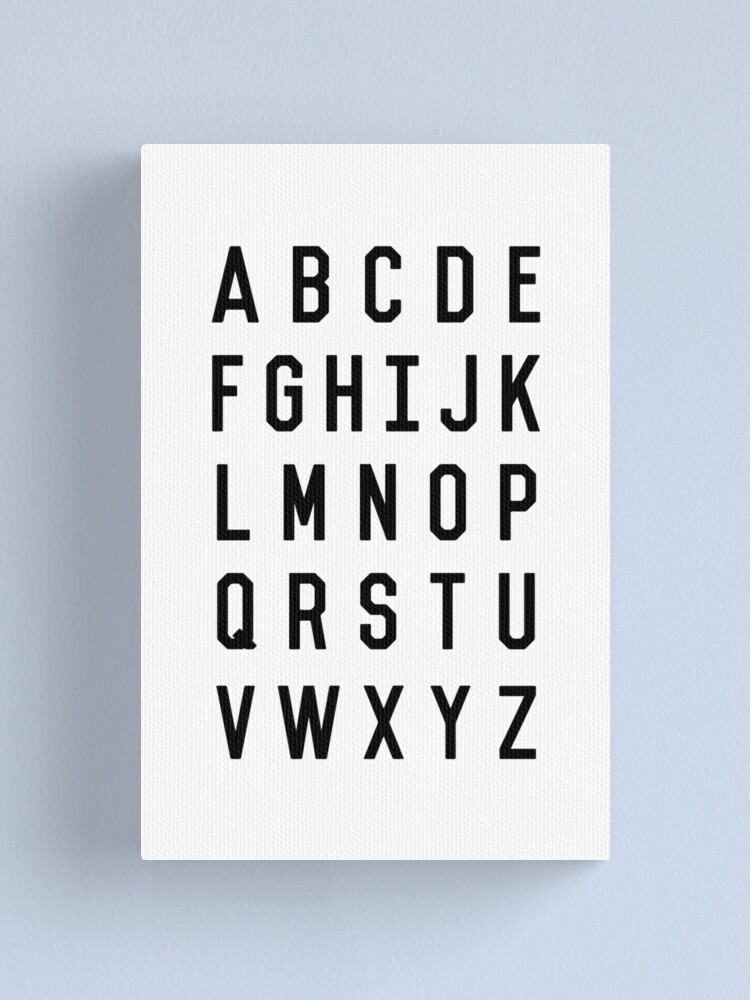The picture portrays a wall with a light blue or powder blue color, featuring a framed poster or art piece with a white rectangular background and no frame. This wall art displays the English alphabet from A to Z, arranged in black, capitalized, sans-serif fonts that appear very geometric and modern. The letters are distributed in five rows, each typically containing five letters, but the second row has six letters to accommodate the entire 26 letters of the alphabet. The overall design is reminiscent of an eye chart used for vision tests due to its clear, easy-to-read, block-style text.